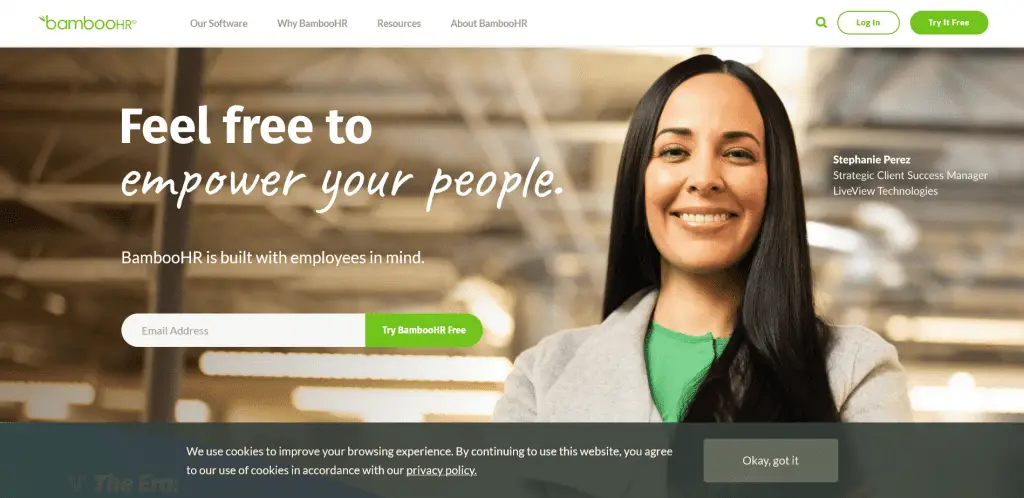The advertisement from the website features the BambooHR logo prominently in green letters at the upper left corner. To the right, menu options are displayed in grey lettering, including "Our Software," "Why BambooHR," "Resources," and "About BambooHR." On the far right of the header, there is a login button, a green "Try it for Free" button, and a search icon.

Below this header, there is a large rectangular image of a woman with dark hair, wearing a green blouse and a light grey coat or sweatshirt. To her left, text reads, "Feel Free to Empower Your People," followed by a subheading that says, "BambooHR is built with employees in mind." Beneath this text, there is a white email address input box with an adjacent green button that says, "Try BambooHR Free." 

To the left of the woman, there is a designation that reads, "Stephanie Perez, Strategic Client Success Manager, Live View Technologies."

At the bottom of the advertisement, there is a dark grey bar with white text that states, "We Use Cookies to Improve Your Browsing Experience. By continuing to use this website, you agree to our use of cookies in accordance with our privacy policy." There is also a button to the right of this statement that says, "OK, Got It."